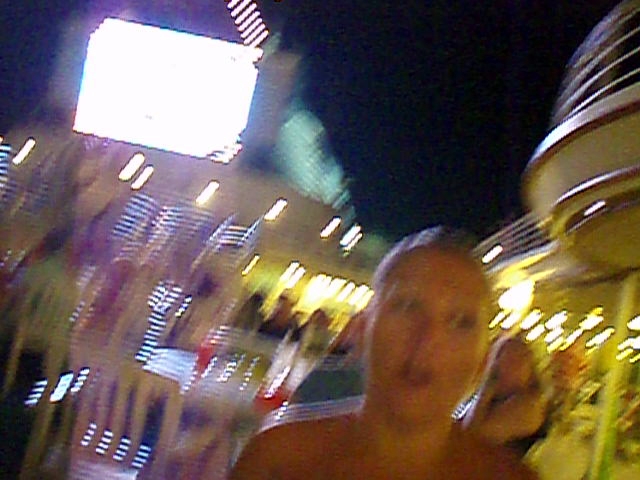In this intriguing and atmospheric image, the blurriness adds an element of mystery, making it challenging to pinpoint the exact setting. It appears to be either a nightclub or a restaurant, potentially located outdoors in a vibrant locale such as Florida, California, the Caribbean, or even a cruise ship. The focal point is a girl with her blonde hair pulled back, wearing either a strapless bikini, shirt, or dress. Her presence adds a lively touch to the scene. Despite the out-of-focus background, you can make out some white chairs, tables, a couple of red cups, and a group of people sitting together. The more you examine the image, the more details emerge, providing subtle clues that hint towards the lively, social environment it captures.